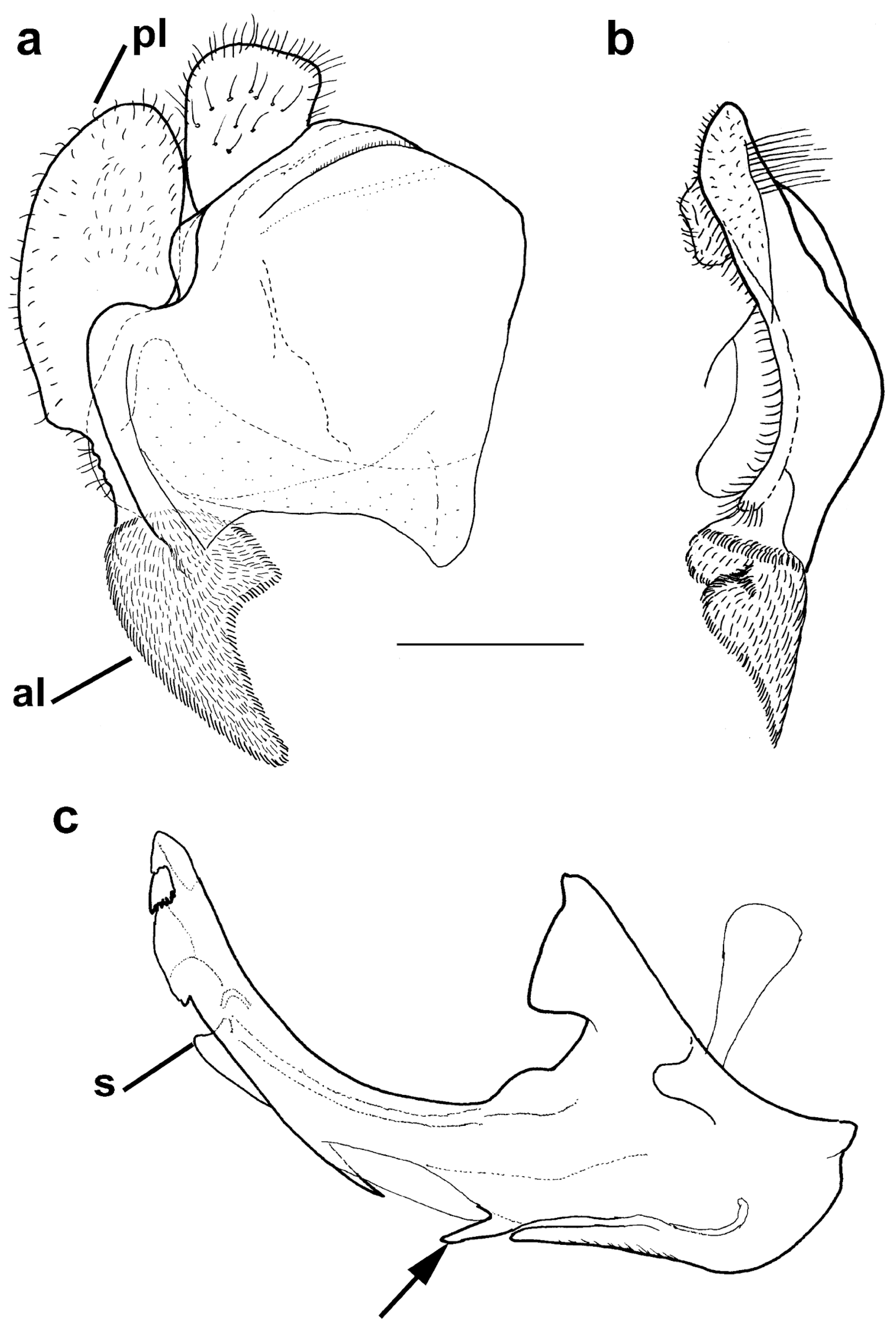The black and white illustration is a detailed anatomical diagram featuring three distinct organic structures, each marked with letters such as A, B, C, P, L, S, and others. Each structure is depicted in black ink, with meticulous cross-hatching and intricate details that could represent bones and flesh. Arrows with labels like PL, AL, and S point to specific parts of these structures. The rightmost structure, labeled with C, resembles a rhinoceros horn adorned with tooth-like protrusions. The middle structure, indicated as B, has a fish-like form with whiskers at the top and a tail featuring similar appendages. The left structure, marked as A, appears triangular with a roundish shape at the top and an elongated section on the left, also sprouting whisker or cilia-like projections. The entire illustration is very thorough, using detailed line work to highlight the organic and possibly anatomical nature of the subjects.